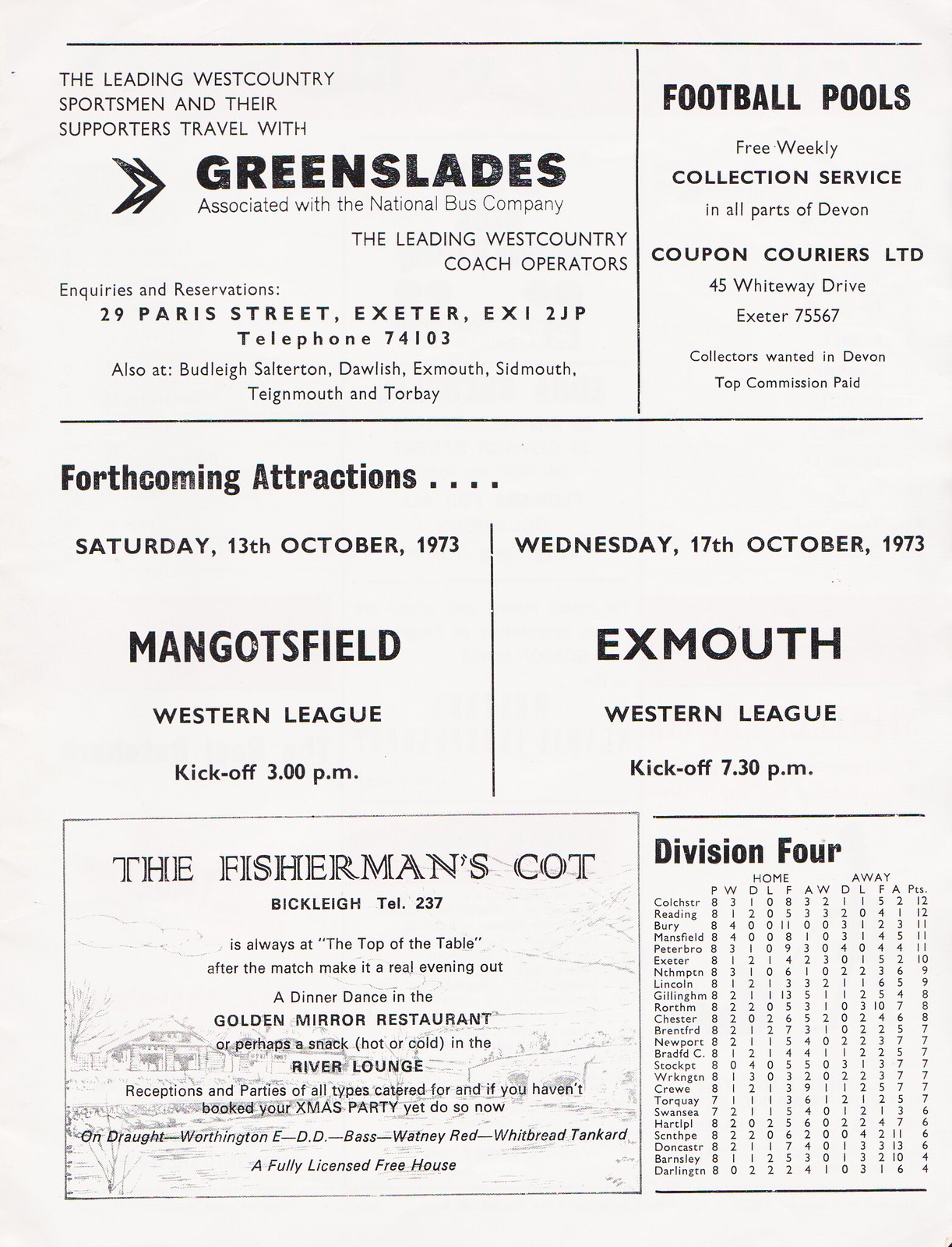This is an image of a printed poster on white paper with black text. It consists of several sections that provide advertisements and football-related information. 

At the upper left is an ad for Green Slades, associated with the National Bus Company, which promotes itself as the leading West Country coach operator. It mentions their service locations in Exeter, Dawlish, Exmouth, Stevemouth, Tegnamouth, and Torbay and provides details for inquiries and reservations at 29 Paris Street, Exeter, EX1, 2JP, with the telephone number 74103.

The upper right section contains an advertisement for a football pool service conducted by Coupon Couriers Ltd, located at 45 Whiteway Drive, Exeter, with the telephone number 75567. They offer a free weekly collection service for football pools in all parts of Devon and are seeking collectors with a promise of top commissions.

In the center, under the heading "Forthcoming Attractions," the poster lists two football matches: one at Mangots Field on Saturday, October 13, 1973, with a Western League kickoff at 3 p.m., and another in Exmouth on Wednesday, October 17, 1973, with a Western League kickoff at 7:30 p.m.

The lower left corner features an advertisement for The Fisherman's Cot restaurant, while the lower right-hand section displays the standings for Division IV football teams.